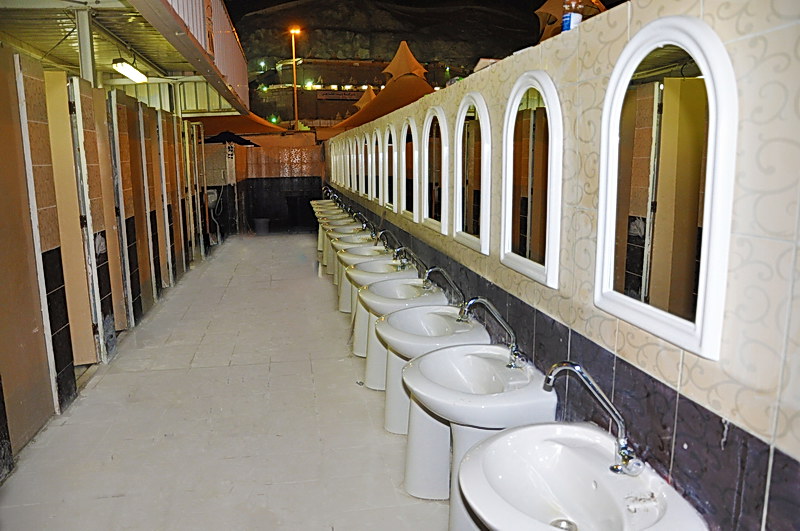This image captures a sprawling commercial bathroom, seemingly part of a stadium or a large public venue. Dominating the right wall is an extensive line-up of approximately 15 to 20 white pedestal sinks, each paired with a tall, stainless steel arched faucet. Above each sink, there are white mirrors with a distinct arched, tunnel-like design. The space has an unexpected feature: an open ceiling that reveals a skyline and distant buildings, giving the entire setup an outdoor feel despite being indoors. The left side of the room features a series of brown stall doors, likely housing the toilets, set against walls adorned with a mix of brown and black tiles. The back wall stands out with its brick-colored and black tiling. The overall ambiance is clean and modern, accentuated by the cream-colored floor tiles and strategic ceiling lighting.